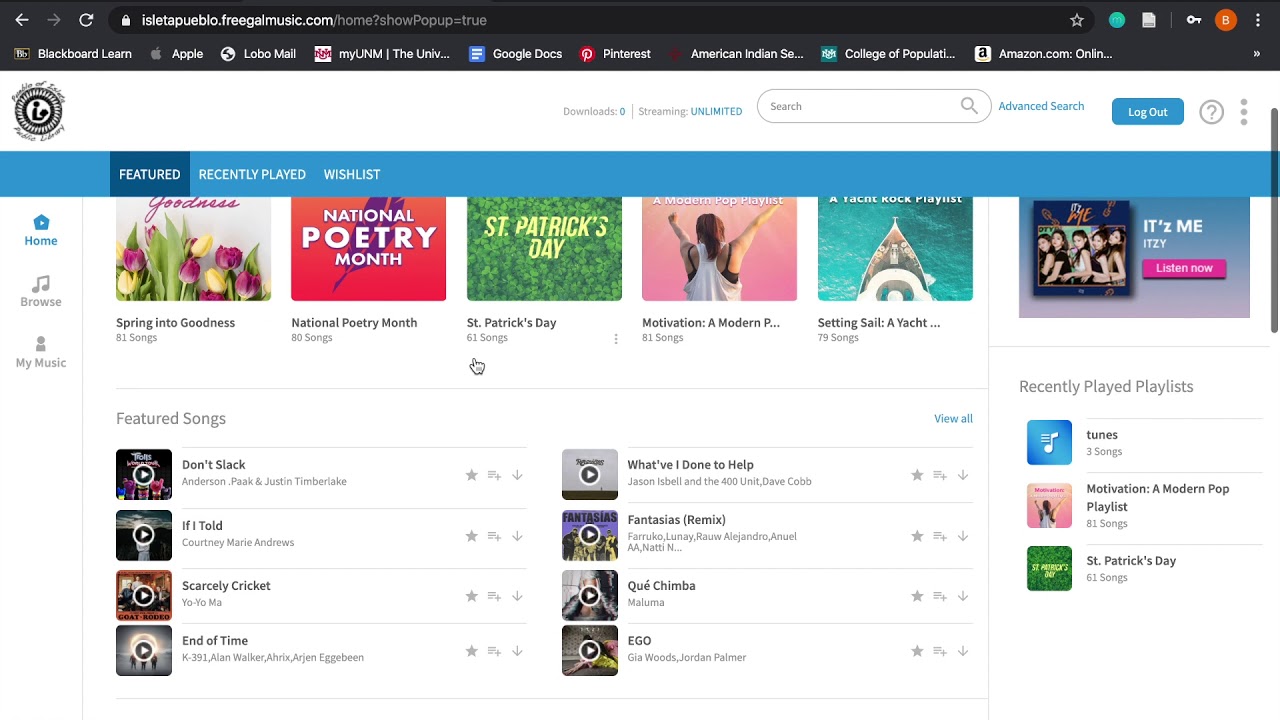The image displays a music web page with the URL isletapureblue.freeganmusic.com. At the top right of the page are several tabs: "Download" (indicated as zero), "Streaming Unlimited," a search box, an "Advanced Search" button, and a blue "Logout" button.

On the left sidebar, there are multiple navigation tabs including "Featured," "Recently Played," and "Wishlist," all written in white on a blue background. The "Featured" tab is highlighted and tabbed in blue. Additional navigation options below these tabs include "Home," "Browser," and "My Music," with "Home" highlighted in blue while "Browser" and "My Music" are grey.

Further down the page, curated playlists are listed, such as "Spring Into Goodness" with 81 songs, "National Poetry Month" with 80 songs, "St. Patrick's Day" with 61 songs, "Motivation" with 81 songs, and "Set in Sale" with 79 songs.

At the bottom of the page, featured songs are displayed in two columns. The left column includes:
1. "Don't Slag"
2. "If I Told" by Courtney Marie Andrews
3. "Ghastly Cricket" by Yo-Yo M.A.
4. "End of Time" by K391 and Alan Walker

The right column includes:
1. "What Have I Done To Help" by Jason Isbell
2. "Fantasias Remix" by Farruko
3. "Kew Chimba" by Maluma
4. "Eagle" by Jordan Palmer

To the right of these featured songs is an advert at the top right corner displaying "It's Me" by E.T., with a pink highlight and the message "Listen Now."

At the bottom of the right sidebar, there is a "Recently Played" playlist section featuring three songs, followed by a "Motivation" modern pop playlist with 81 songs, and a "St. Patrick's Day" playlist with 61 songs.